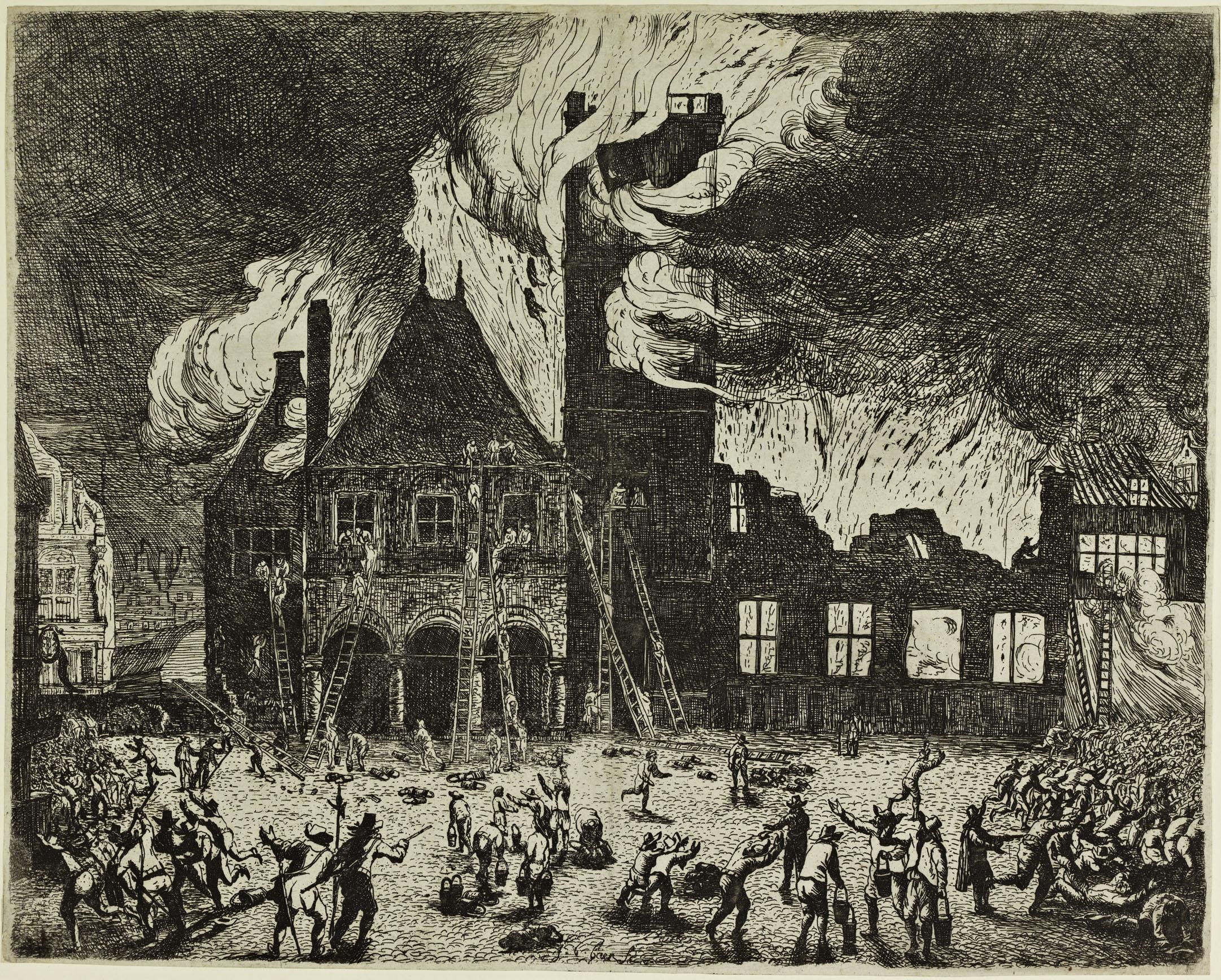This black and white etching captures a harrowing nighttime scene of a large-scale fire engulfing a series of buildings in what appears to be a residential neighborhood, possibly referencing a historical event like the Chicago Fire. The artwork is rendered with pencil, giving it a monochromatic and somber tone. Five buildings are fully consumed by roaring flames that shoot dramatically into the sky, casting an eerie glow over the chaotic scene. Ladders lean against the sides of the buildings, and people swarm the streets, staring in horror and panic. Some are depicted with their arms up, suggesting helplessness, while others seem to be attempting futile efforts to combat the blaze. The smoke billows ominously above, adding to the tragic and catastrophic atmosphere of the city being consumed by fire.